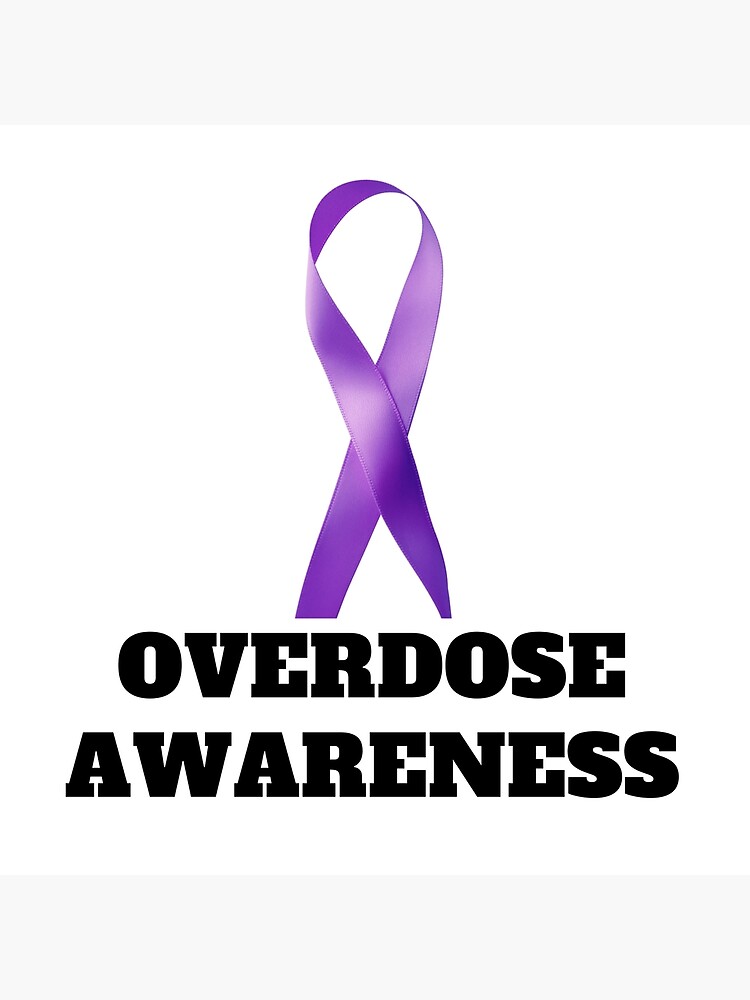The image portrays a purple ribbon, similar in shape to the pink breast cancer awareness ribbon, with a loop at the top and folded over itself. This ribbon is set against a plain white background. Below the ribbon, in bold black serif font, are the words "Overdose Awareness." Additionally, there are light blue bars at the top and bottom of the image, providing a border.